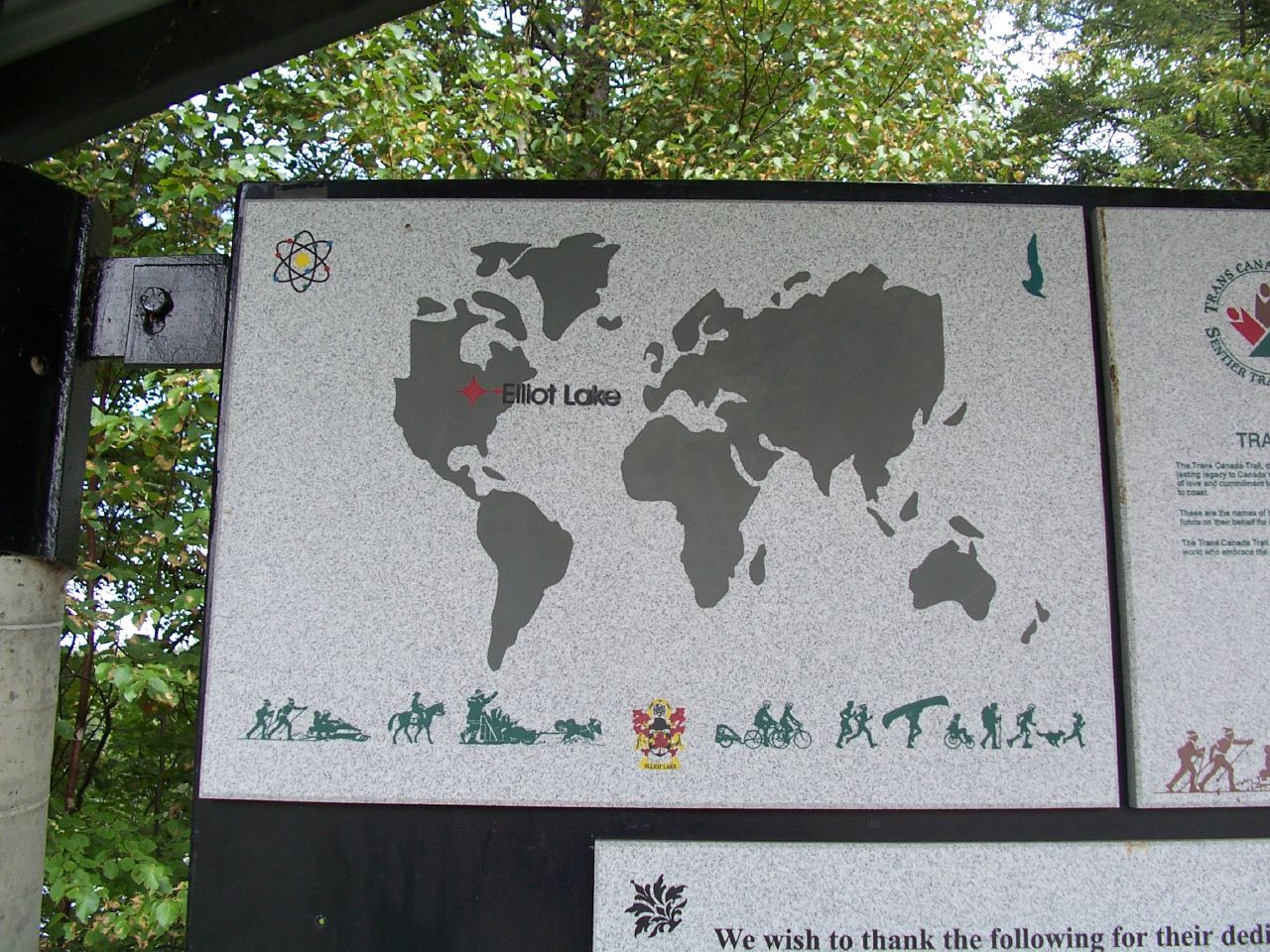The image depicts an outdoor stone sign mounted on a metal plaque, secured onto a concrete slab with bolts. The background is filled with lush green trees. The sign features a world map in gray shades with a distinct red star marking the location of Elliot Lake in North America. In the top corners, the sign is adorned with two symbols: a bird emblem on the right and a flower-like logo made of overlapping circles on the left.

The map is complemented by a variety of colored accents, including touches of red, blue, green, and yellow. Below the map, a series of green silhouette drawings illustrate various recreational activities. These include people cross-country skiing, snowmobiling, horseback riding, dog sledding, bicycling, running, carrying a canoe, using a wheelchair, hiking with a stick, rollerblading, and running with a dog. Additional slabs with mostly unreadable text flank the sign on the right and below.